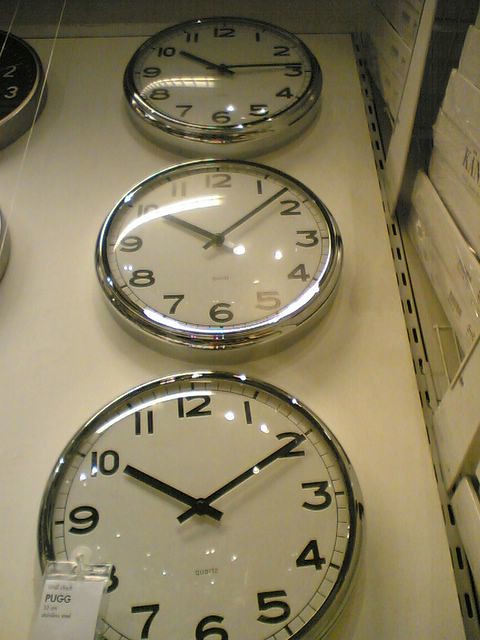The image depicts a display area in what appears to be an Ikea store, featuring three simple, modern wall clocks arranged vertically in a column against a plain white wall. Each clock has a white face with black numbers and hands, encased in a metallic chrome frame. A small, rectangular label affixed to the bottom clock reads "PUGG." To the right of the display, shelves hold boxes likely containing the clock models, while to the left, a portion of another clock with a black background and a similar chrome frame is visible. The overall photo has a dark, yellowish tint, with bright lights causing reflections on the glass faces of the clocks. The times displayed on the clocks vary slightly, showing 10:15, 10:08, and 10:10, respectively.